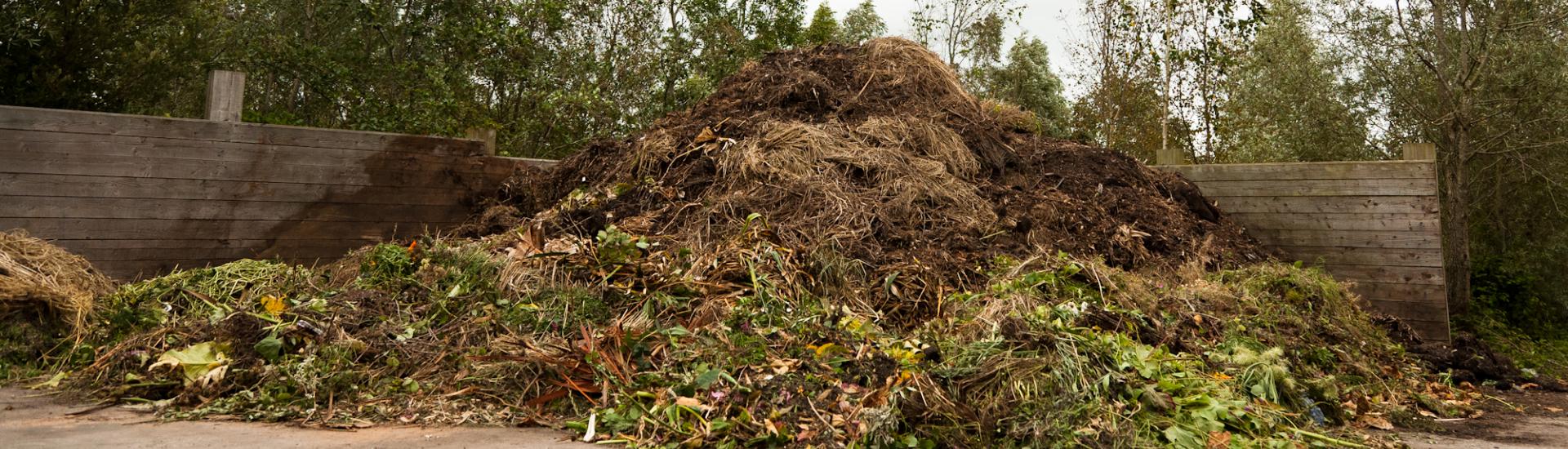In front of a forested area and a stone wall with multiple towering pillars, a massive compost pile is situated, creating a vivid scene. The wall forms an L-shape, with its stone texture anchoring the compost pile that spans nearly from one corner of the L to the other. Dominating the scene, the compost pile is a mix of dead leaves, plant material, and hay. At the front of the pile, green branches, leaves, and grass are visible, hinting at the fresher additions. As your eyes move towards the middle, patches of old hay are discernible, before reaching the back, where the pile rises high and consists of a combination of manure, old grass clippings, and brush cuttings. The stone wall bears signs of moisture where the compost is pushed up against it, emphasizing the natural recycling process occurring in the pile. The surrounding is lit with daytime light, but an overcast sky suggests a potential for a dreary, cloudy day, as not much sky is visible through the dense foliage behind the wall.